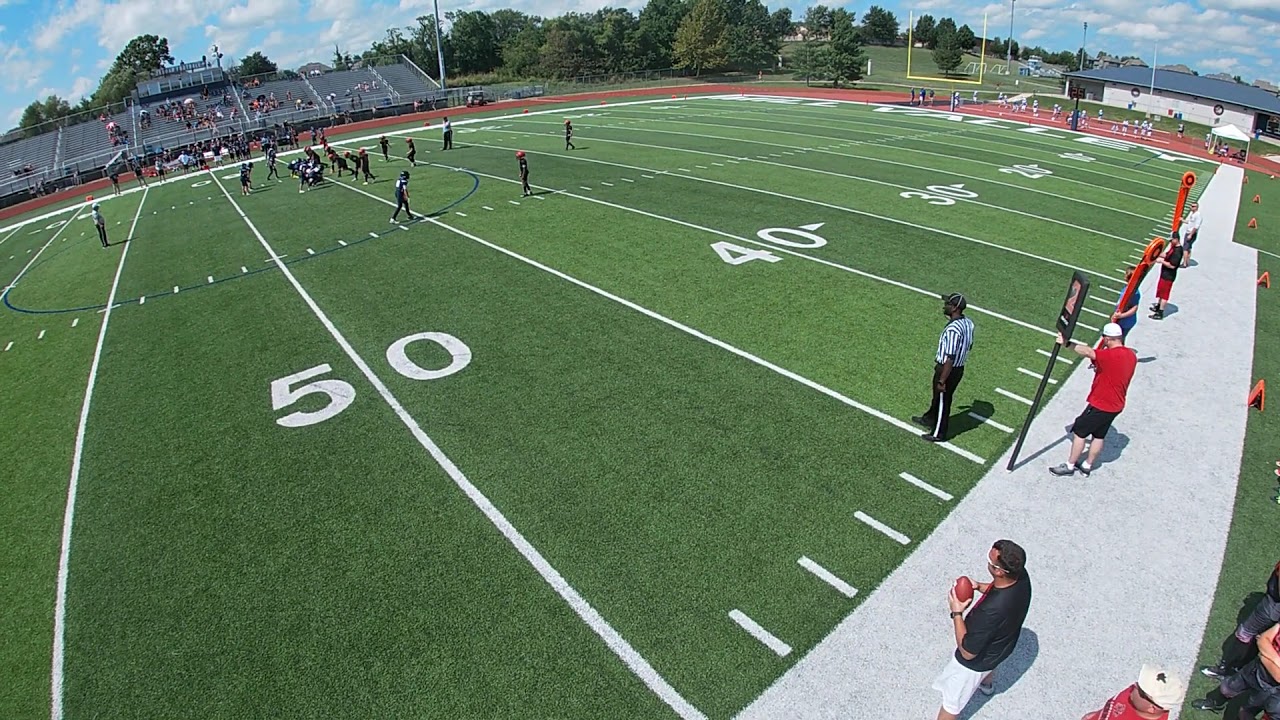This image showcases an outdoor scene of a football field captured from the 50-yard line with a distinctive fisheye lens effect, causing the field lines to curve towards the horizon and making the people on the field appear much smaller and further away than they really are. You can see tiny human figures spread across the field, suggesting a game is in progress, likely involving a youth football team, given their smaller, less athletic appearance, indicating they're probably middle school or high school kids.

The image’s unusual angle hints at it being taken from a high vantage point, possibly via a very long selfie stick or an initial drone lift-off. In the foreground, a referee in a classic striped shirt stands near the white sideline, alongside several men in various colored t-shirts and shorts, with others milling about nearby, possibly coaches or parents.

Towards the upper left, a set of bleachers is visible with sparse attendance. The right-hand side shows additional elements including signs indicating game status—such as “Second Down”—and people holding football gear. On the opposite end, the end zone bears the partially visible name ending in “valley,” perhaps the team or school's name. The backdrop includes trees, a goal post, a running track, and white buildings, with soccer nets and a partly cloudy sky completing the scene.